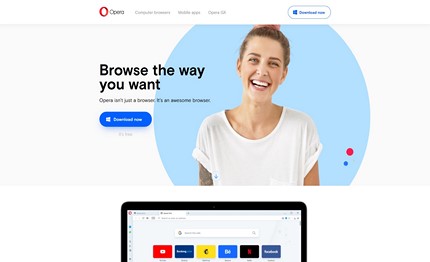The image showcases the landing page for the Opera browser installation. Dominating the center is a large photo of a woman standing in front of a light blue circle, smiling broadly, seemingly pleased with the Opera browser. The tagline "Browse the way you want" is prominent, emphasizing Opera's user-centric design. Below this tagline, a description highlights that Opera isn't just any browser; it’s hailed as an incredible browsing solution.

Beneath the promotional text, there is a noticeable call-to-action button inviting users to "Download for Windows." Adjacent to this, a slightly blurry image depicts a laptop screen with the Opera browser open, providing a glimpse of its interface. Although the image quality is not crystal clear, several recognizable icons on the browser’s homepage hint at quick access to popular websites such as Netflix, Facebook, and YouTube, alongside a few indistinguishable ones.

At the top of the page, another "Download Now" button for Windows Opera is visible, reaffirming the call to action. Additional navigation options are available, including a section about the mobile widget, a Q&A segment, and a tab for company investors. Despite the overall blurriness of the image, the woman’s joyful expression vividly conveys a positive user experience with the Opera browser.